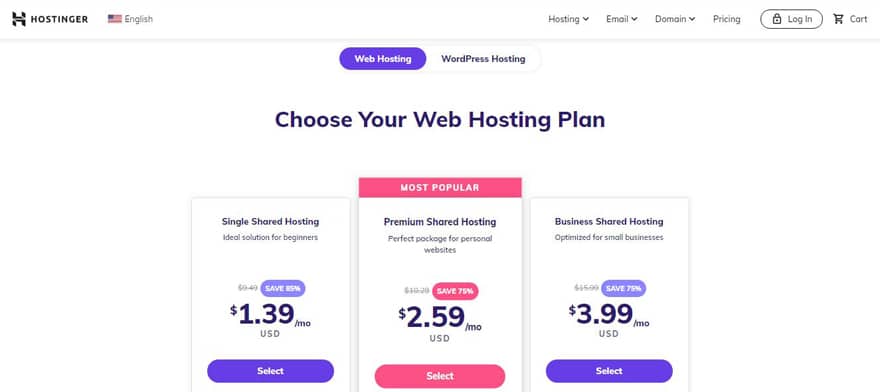This screenshot captures the homepage of Hostinger, a web hosting platform. The top section features a navigation bar with the Hostinger logo, which resembles an "H" and is followed by the word "Hostinger" in bold. Adjacent to the logo, there's an American flag icon signifying the selected language, English. To the right of these elements, the ribbon menu displays the following options: "Hosting" with a dropdown arrow, "Email" with a dropdown arrow, "Domain" with a dropdown arrow, a "Pricing" link, a login button bearing a lock symbol, and a cart icon accompanied by the word "Cart." 

Below this navigation ribbon, a thin gray line separates it from the subsequent section, where two hosting options are presented. The currently selected option is "Web Hosting," with "WordPress Hosting" being the unselected alternative. 

The main headline reads "Choose Your Web Hosting Plan," under which three hosting packages are showcased in distinct boxes:

1. On the left, the "Single Shared Hosting" box is labeled as the "Ideal solution for beginners," offering a substantial discount of roughly 85%, at a promotional price of $1.39 per month. A button labeled "Select" is positioned below.

2. The center box, highlighted as "Most Popular" in pink, features the "Premium Shared Hosting" option, described as the "Perfect package for personal websites." It offers a 75% discount, priced at $2.59 per month. This option also includes a pink "Select" button at the bottom.

3. To the right, the "Business Shared Hosting" box is targeted towards small businesses, also offering a 75% discount, with a price of $3.99 per month. A purple "Select" button is located below this package.

These details encapsulate the content visible in the screenshot, outlining the primary web hosting plans offered by Hostinger.